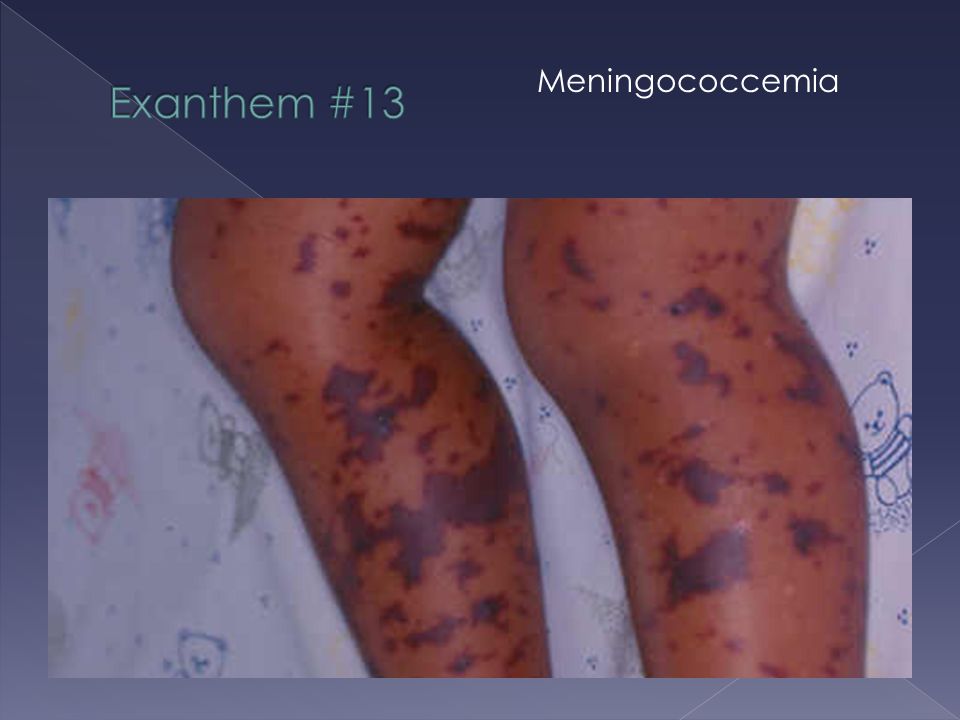The image depicts a medical slide presentation with a background gradient of shades of purple. The main focus of the slide is a close-up photograph of a child's legs, positioned at the bottom of the image, laying on a white bed sheet adorned with colorful teddy bear illustrations. The child's legs are visibly swollen and covered in dark red and brown splotches, indicative of a possible disease. The text on the slide includes "Exanthem number 13" and "Meningococcemia," providing context for the condition being shown. This detailed slide likely serves as part of a medical journal or educational material to demonstrate symptoms of the disease.